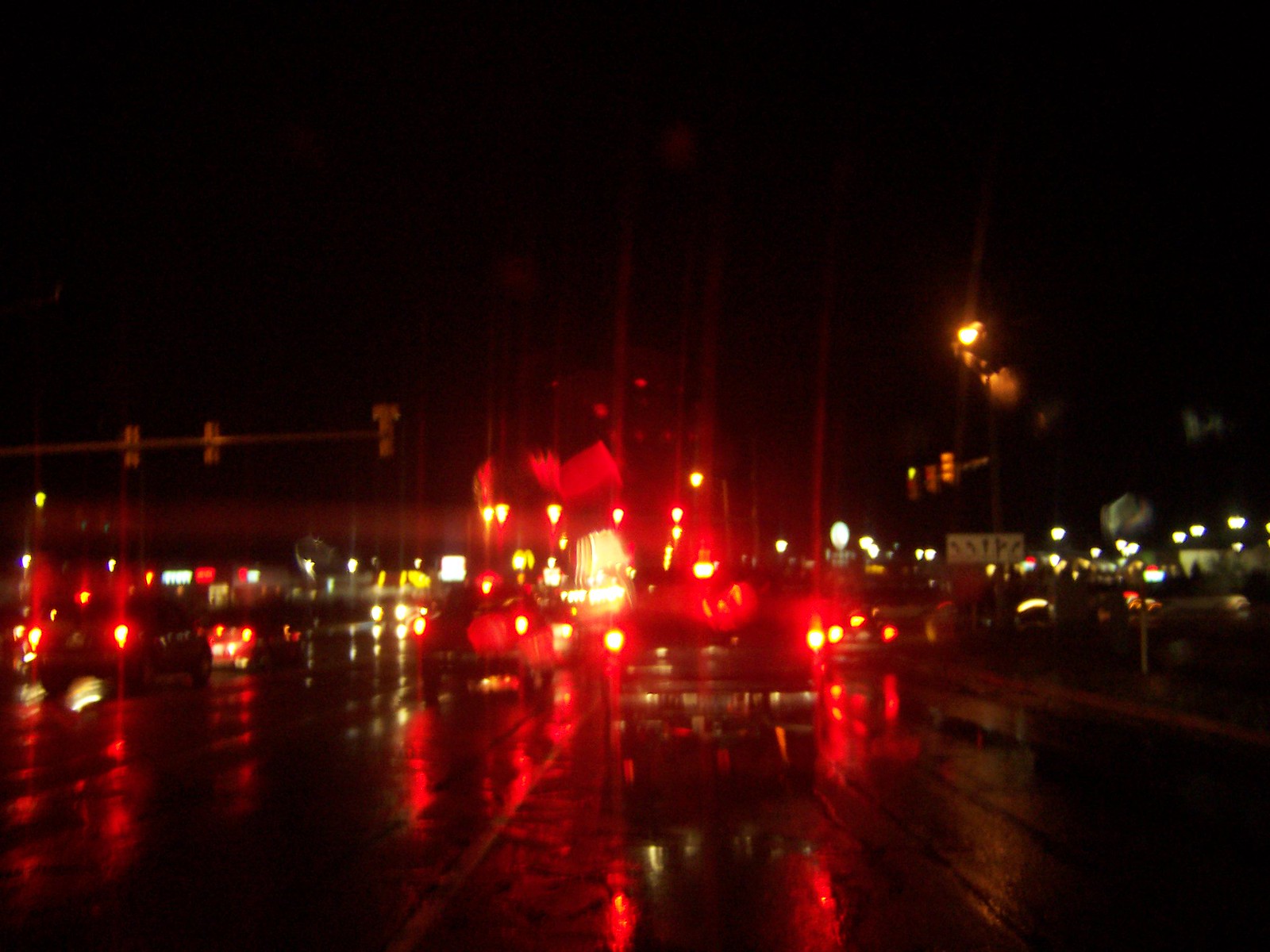In this nighttime photograph of a motorway service stop, possibly a petrol station, the scene is blurred and out-of-focus, creating a vibrant display of colorful lights amidst a rainy backdrop. The wet road, slick with rainwater, reflects these lights, causing red taillights from various vehicles to streak across the pavement with a striking intensity. The image features a collection of vehicles, including a prominent truck with numerous red lights on its cab, accompanied by smaller vehicles whose taillights contribute to the red glow. The black sky is illuminated by a glimpse of the moon overhead and distant store lights, casting white light into the scene. There are several road signs with arrows on the right side of the road and a tall traffic light with a red stop signal on the left. Amidst the flares and reflections, yellow housings and bars of the traffic lights can be discerned. The overall atmosphere is defined by the dark, wet, and busy road, with both natural and artificial lights piercing through the nighttime haze.